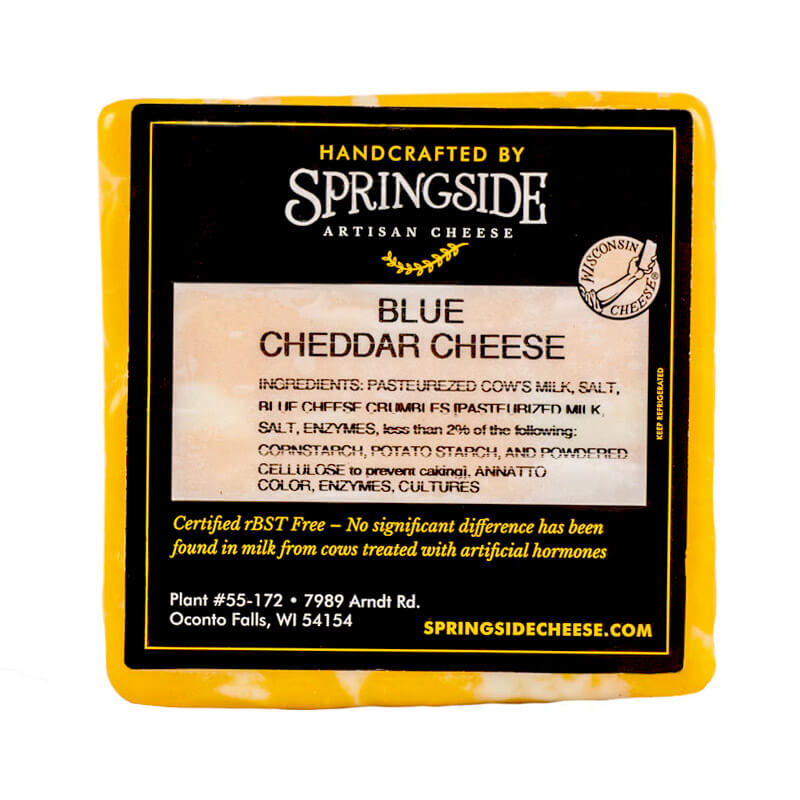This top-down photograph features a square block of marbled orange and white cheddar cheese, with slightly curved sides and corners, typical of a store-bought cheese package. The cheese is wrapped in a shiny plastic, and prominently displays a full square black label on the front. The label is detailed with yellow, white, and black print. At the top, it reads, "Handcrafted by Springside Artisan Cheese," followed by the type, "Blue Cheddar Cheese." The ingredients listed are pasteurized cow's milk, salt, blue cheese crumbs, enzymes, corn starch, potato starch, and powdered cellulose to prevent caking. It is also noted as being RBST-free, with an explanation that no significant difference has been found in milk from cows treated with artificial hormones. The manufacturing details list "Plant 55-172, 7989 Arndt Road, Oconto Falls, Wisconsin, 54154." The label also includes a web address at the bottom right corner that reads "springsidecheese.com."